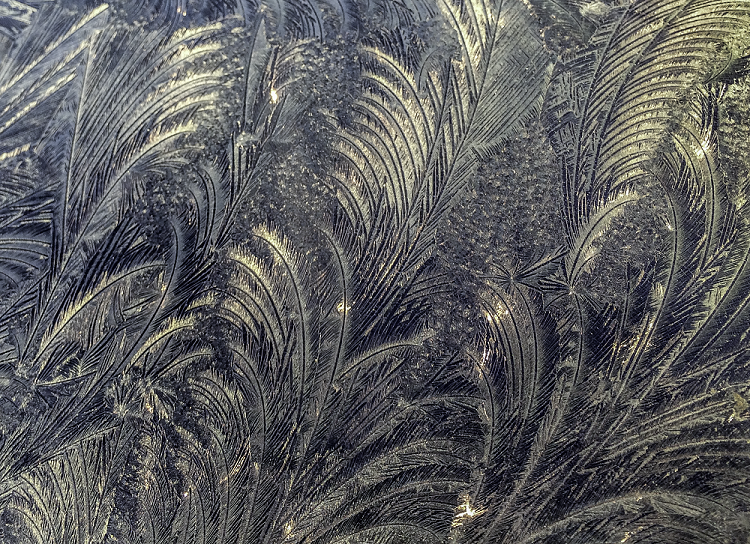This is a highly detailed, monochromatic, hand-drawn sketch of an outdoor scene dominated by tall, elongated palm fronds or potentially tall grasses. The entire composition is filled with these fronds, which appear to be swaying to the right, likely suggesting the presence of a gentle breeze. The drawing exhibits meticulous shading, possibly using charcoal or pencil, which adds depth and texture to the dense, abundant foliage. The interplay of light and shadow is evident, with small areas of white breaking through the otherwise dark sketch, reminiscent of sunlight filtering through the fronds. The sketch captures a close-up view, focusing on the midsection of the fronds or grasses, without showing their roots or tops. The long, thick stems lead into billowing smaller leaves, creating a rich, dynamic scene that evokes the natural movement and intricate beauty of a jungle or dense grassland.